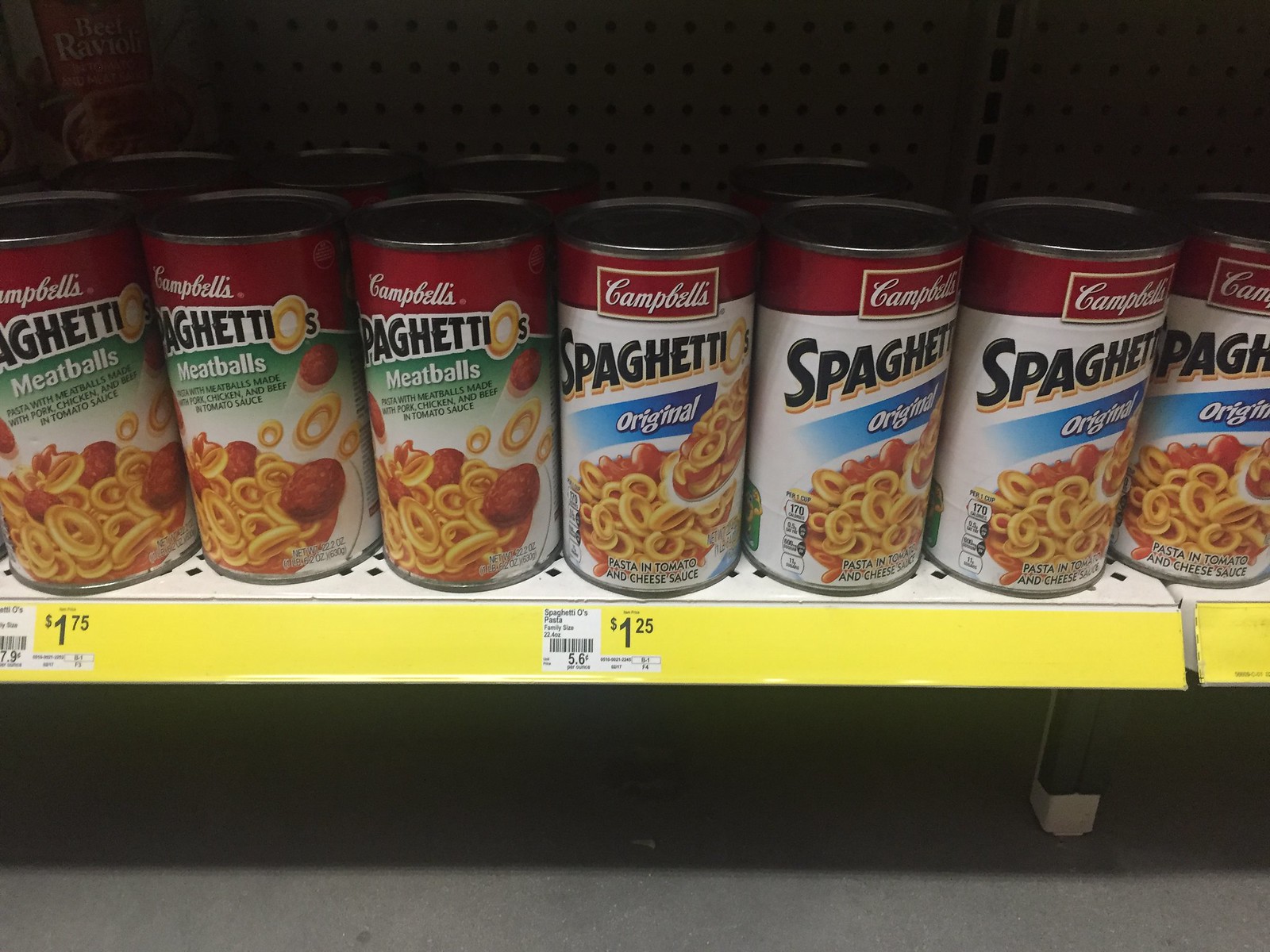This photograph captures a grocery store shelf displaying various versions of Campbell's SpaghettiOs. The top of each can prominently features the Campbell's logo. On the left side of the shelf, there are three cans of SpaghettiOs with Meatballs, each priced at $1.75. On the right side, there are four cans of Original SpaghettiOs, each priced at $1.25. In total, there are seven cans of SpaghettiOs, divided between six cans of the meatball variety and five cans of the original. The cans are arranged in two rows, with one row in front and another behind, indicating a well-stocked shelf. The price difference suggests an additional cost of 50 cents for the meatball variety. Notably, there seems to be a higher number of Original SpaghettiOs, hinting at better sales for this variant.